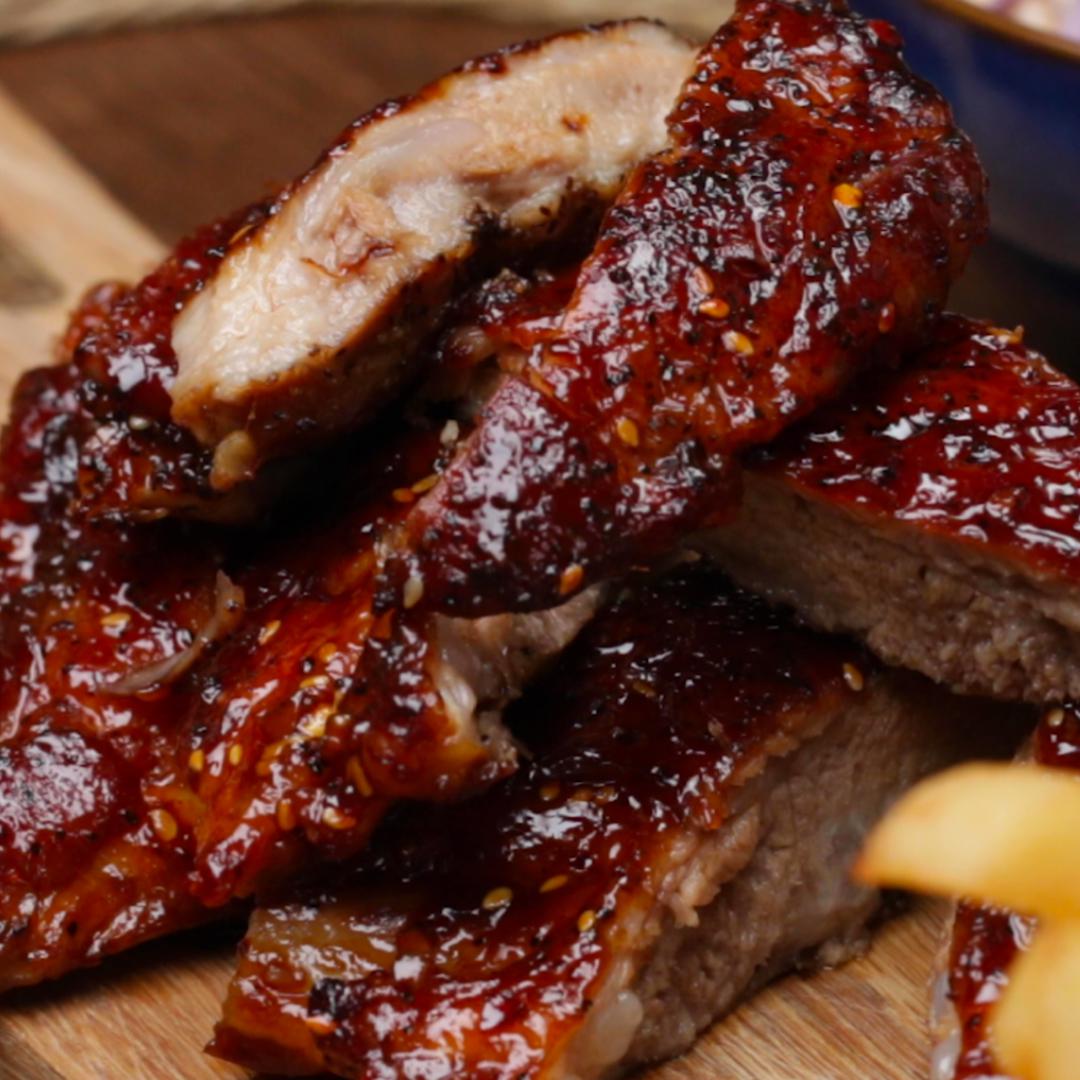The photograph captures a tantalizing display of what appears to be Chinese barbecue ribs, masterfully arranged and covered in a rich, reddish barbecue sauce. The ribs, stacked unevenly, exhibit a variety of textures and colors, hinting at different stages of the barbecue process. Each piece showcases a darker, almost pecan or mahogany wood char, with some areas boasting a delicious black crisp. The side views of the ribs reveal the grain of the meat, suggesting a juicy and tender interior.

In the bottom right corner of the image, a hint of a yellow object—possibly a lemon or squash—adds a contrasting splash of color. This vibrant detail stands out against the backdrop of a wooden surface, which could be a rustic tabletop or cutting board, enhancing the earthy and hearty presentation. The wood varies in tone, with lighter sections juxtaposed against richer, darker hues, framing the savory ribs in an inviting, natural setting.